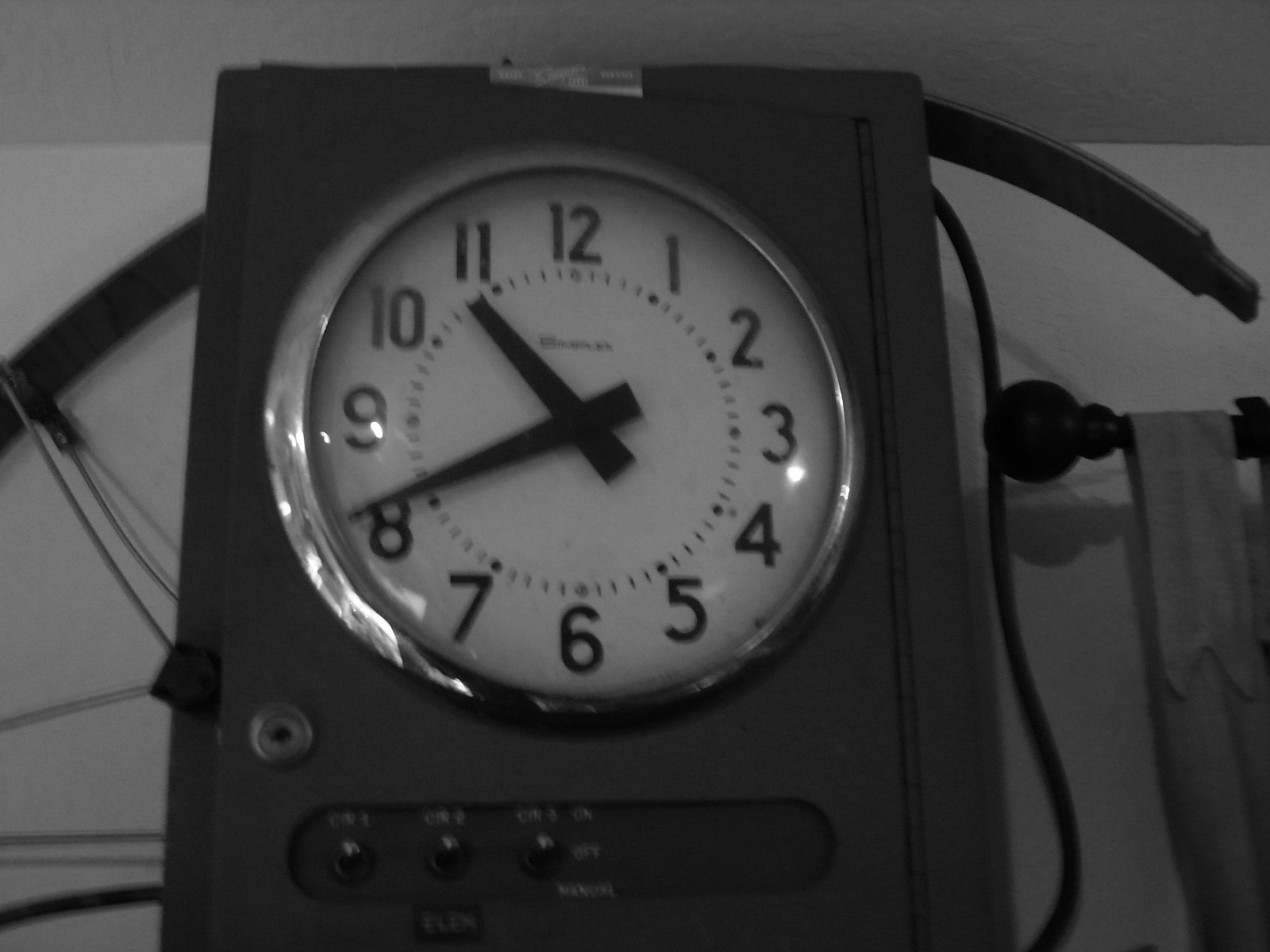This is a close-up photograph of a metal clock with an intricate design. The clock, featuring a robust gray box-like base, is captured in fine detail. Positioned on the right side, a drapery rod with a round black newel is partially visible, supporting white panel drapes hung by tabs. The clock's face, large and encircled by a sleek silver ring, stands out against the white background. Prominent black hour and minute hands point towards bold black numerals, with dots and hash marks demarcating 12-minute intervals around the clock's circumference. Below the clock face, three switches arranged linearly provide functional control, while a metallic keyhole on the left side adds a hint of vintage charm. Two distinctive metal arm-like structures elevate on either side of the clock, contributing to its unique aesthetic.